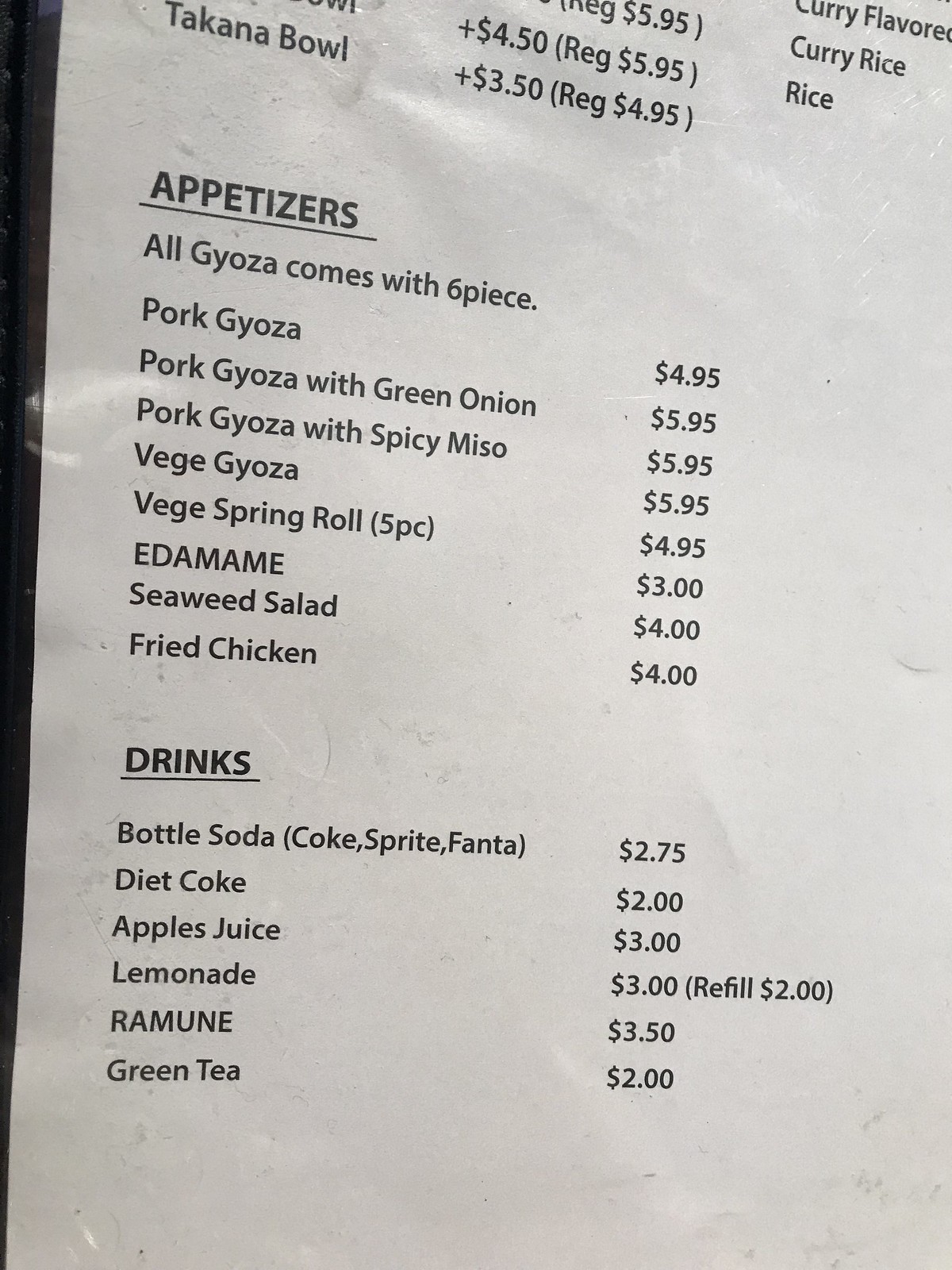This photograph captures a menu printed on solid white paper with black lettering. The top section of the menu is cut off, making only part of some dishes and prices visible, such as a Takana bowl, some curry dishes, and rice.

The middle part of the menu is clearly visible. The heading "Appetizers" is printed in bold with a horizontal line beneath it. This section lists various appetizers, noting that all gyoza come in six pieces. The gyoza options are followed by other appetizers like edamame, seaweed salad, and fried chicken, each accompanied by their respective prices aligned with dollar signs on the right.

Below the appetizers, there's a section for drinks, where the word "Drinks" is also bolded with a horizontal line underneath. This section includes bottled sodas like Coke, Sprite, and Fanta, priced at $2.75. Additional drink options include Diet Coke, "Apples Juice" (notably misspelled with an extra 's'), lemonade (with an indication that refills are charged), Ramune, and green tea.